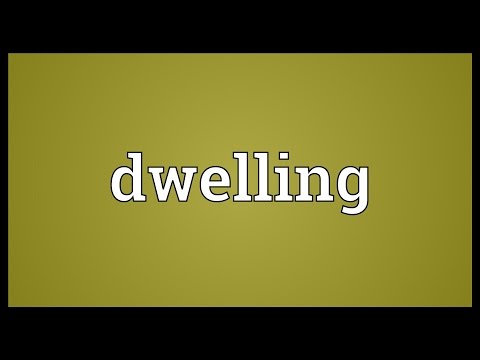The image features a black rectangular background, closer to a square in its proportions, with a thinner black border on its vertical sides and a much thicker one on its horizontal sides. Centered within this black frame is a rectangular olive-colored box. Within this olive rectangle, the word "dwelling" is meticulously centered and written in all lowercase white letters, each outlined in black. The letters are evenly spaced, more so than typical text, enhancing the emphasis on the word. The corners of both the olive box and the black border are pointed, and the smooth surfaces are devoid of any additional lines or textures. The design's simplicity and precision draw attention to the word "dwelling," making it the focal point of the image.